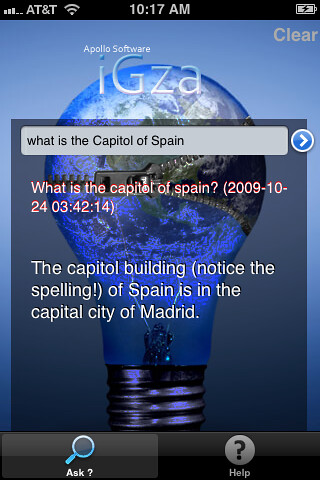The image is a detailed screenshot taken from an iOS device, displaying an app interface at the top. The screen shows the AT&T service with three bars, a Wi-Fi connection, the time as 10:17 a.m., and a battery symbol. The app in view is identified as "Apollo Software IGZA". Taking up the entire screen is a central element where a user has typed in the question, "What is the capital of Spain?" This question appears twice in the screenshot: once in a white search bar with black text, and again below it in a white font with a red outline. Below this, it provides an answer stating, "The capital of Spain is the capital city of Madrid," although it notes the spelling of "Spain". Amid this text, the date "2009, 10, 24" and the number "3, 42, 14" are also visible. The background of the screenshot features a light bulb with a zipper in the center, symbolizing the lock screen. Additional elements include a tab for "Ask" and another for "Help" at the bottom of the screen. The predominant colors used in the interface are black, white, blue, gray, and red.